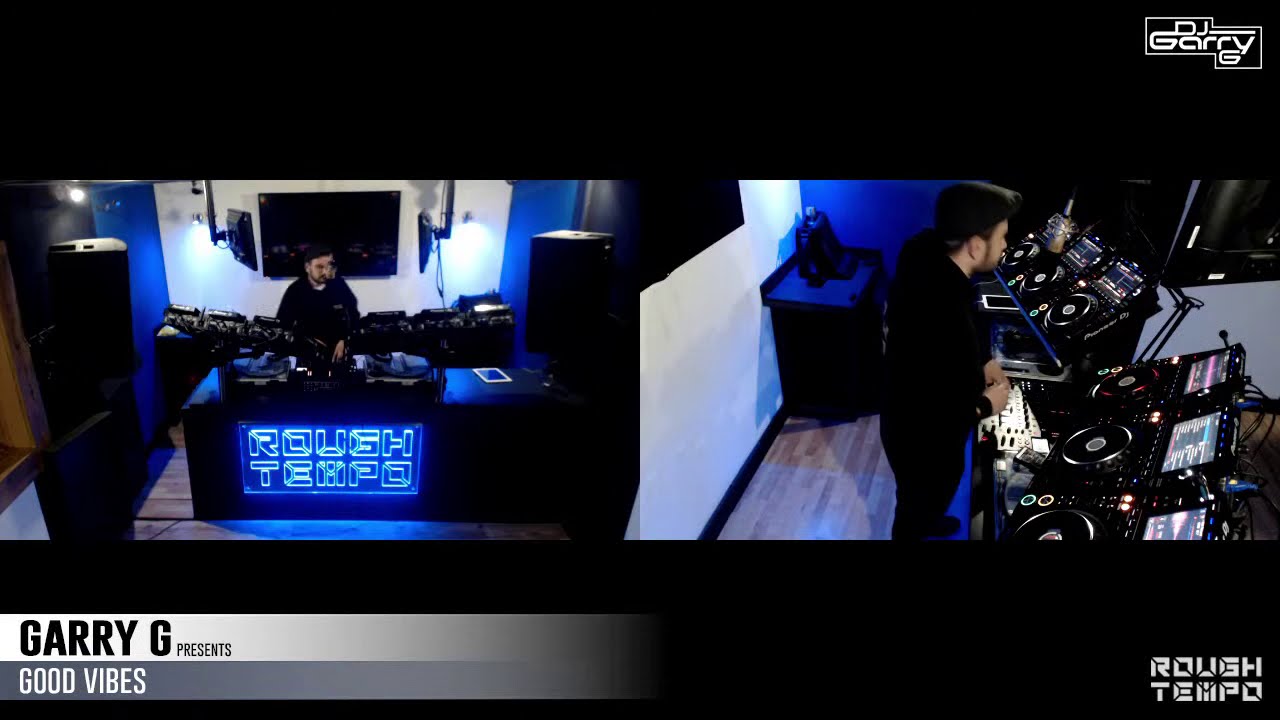This image collage showcases DJ Gary G performing in his DJ setup from two distinct angles. The left image provides a frontal and slightly elevated view, capturing DJ Gary G behind his DJ station, which is equipped with a variety of spin tables, digital screens, and an array of light-up buttons and dials. The setup includes a black table with a neon blue sign reading "Rough Tempo" on the front, and speakers set up on either side. The background features a white wall with a black TV screen flanked by two monitors. 

The right image offers a side view from DJ Gary G's right, giving a clearer glimpse of the intricate equipment he uses, including three monitors on each side of his DJ setup. This angle also showcases the wooden floor beneath him. Both images highlight a well-lit room with walls adorned with lights, adding to the ambiance.

Text adorns the collage: "DJ Gary G" in white text on a black background at the upper right, "Rough Tempo" at the lower right, and "Gary G Presents Good Vibes" in black and white text on a gray banner in the lower left. This detailed setup reflects DJ Gary G's immersive Rough Tempo scene, emphasizing his focus and the intricate design of his performing space.